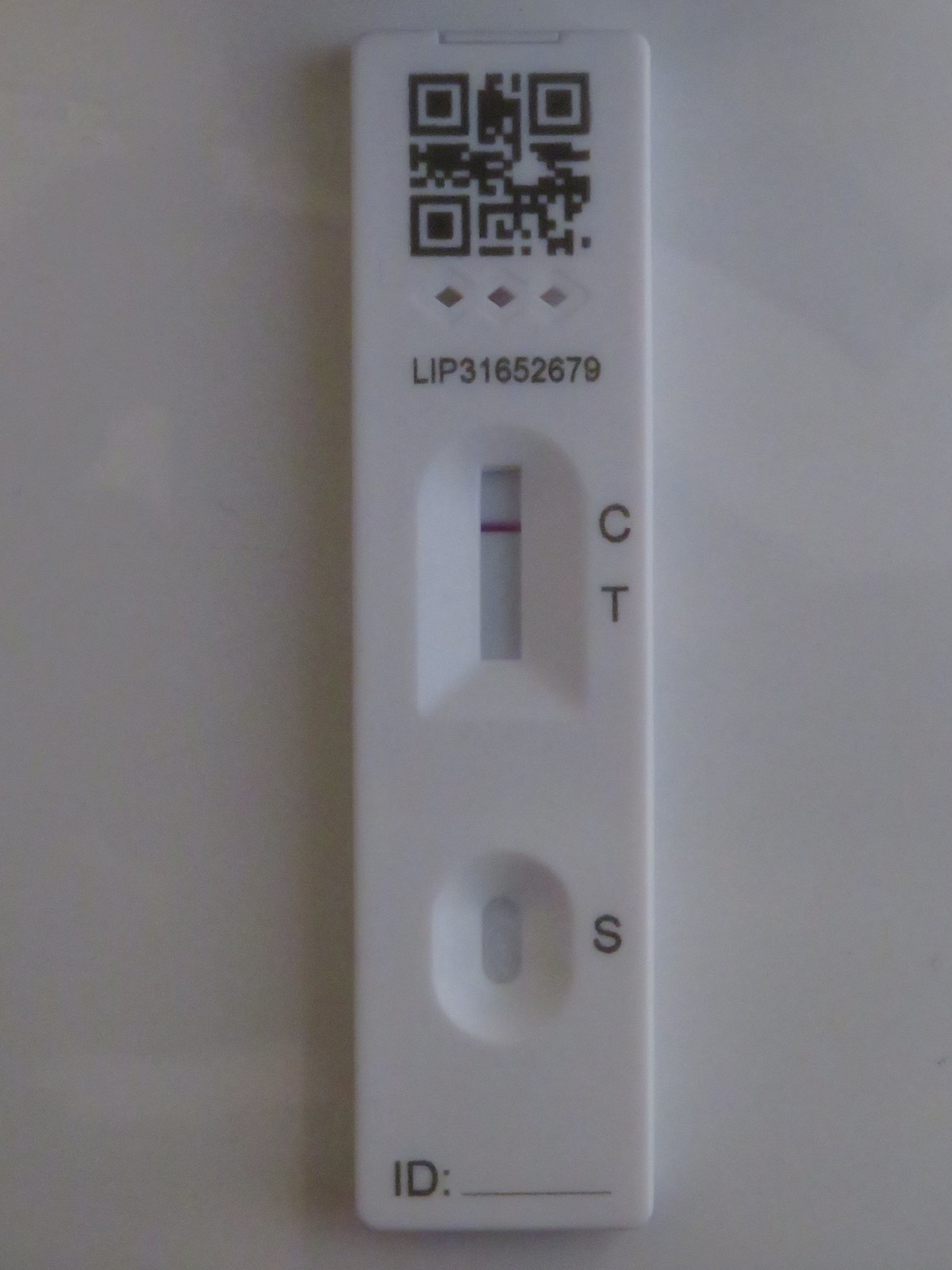This is an image showcasing a white COVID-19 test kit against a white background. At the top of the test, etched in bold, is the identification number "LIP 31652679." Immediately below this, the test features a rectangular area with a purple horizontal line aligned next to the letter "C," signifying the control indicator. Beneath this, there's an ovular indentation adjacent to the letter "S," marking the sample application spot. Further down, the label "ID" is prominently displayed in capital letters beside a blank line intended for additional identification details. The overall design and structural details of the test kit are clear and precise, highlighting its functionality and layout.